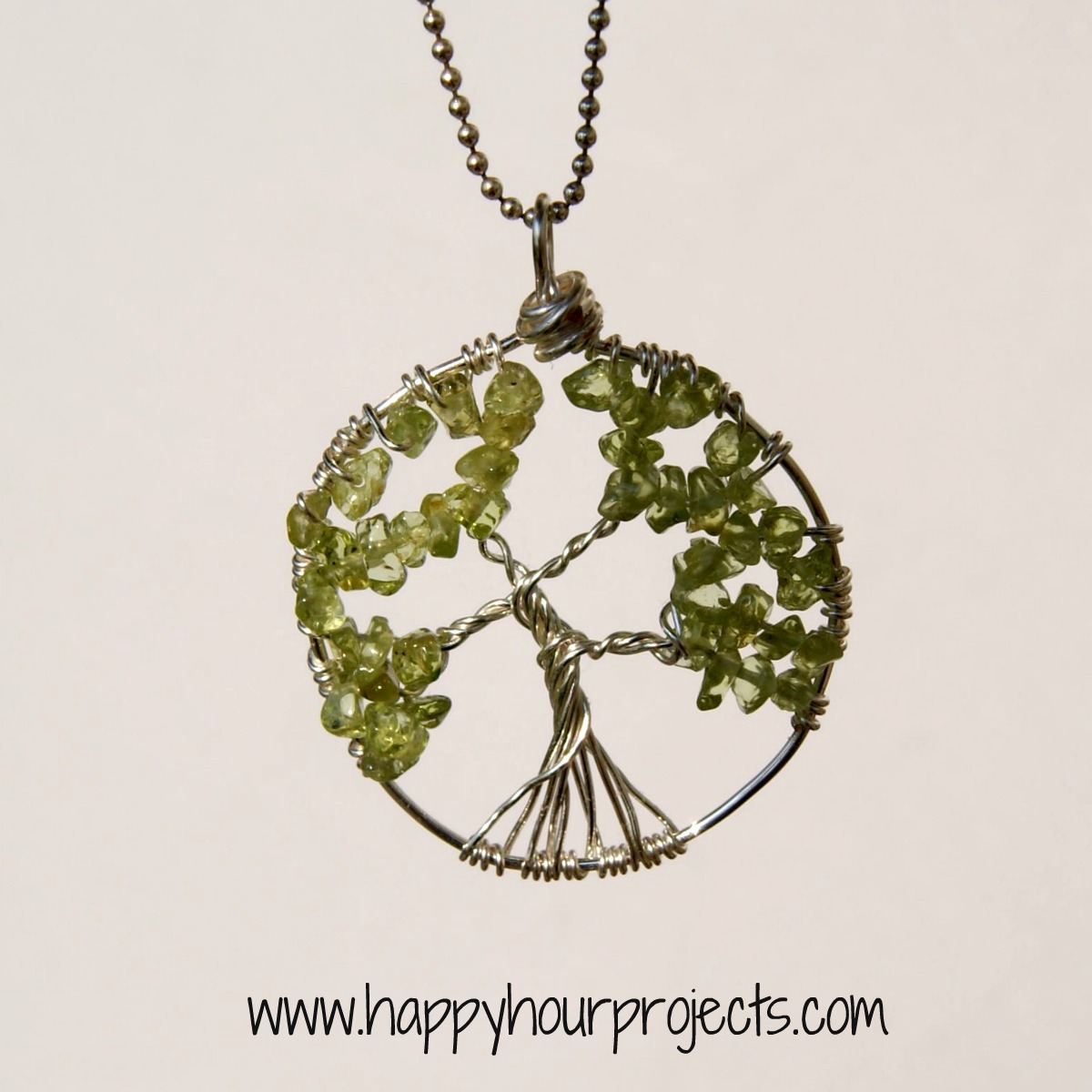The picture features a neatly centered, handcrafted necklace displayed against a predominantly pale off-white background with subtle gray and brown tones. The focal point of the image is a delicate silver ball chain, reminiscent of those used for dog tags, which curves gently at the top. This chain suspends a distinctive circular pendant, approximately 2 inches in diameter, intricately formed from tarnished silver wire. The pendant hosts an artistically wire-wrapped tree design, its branches adorned with light green glass beads. This meticulous craftsmanship is emphasized as the sole object in the image, surrounded by elements in muted hues of light gray, dark gray, silver, green, black, and white. The serene simplicity and symmetry of the presentation suggest it might be a part of an advertisement for the jewelry, as indicated by the neatly printed text at the bottom: www.happyhourprojects.com.